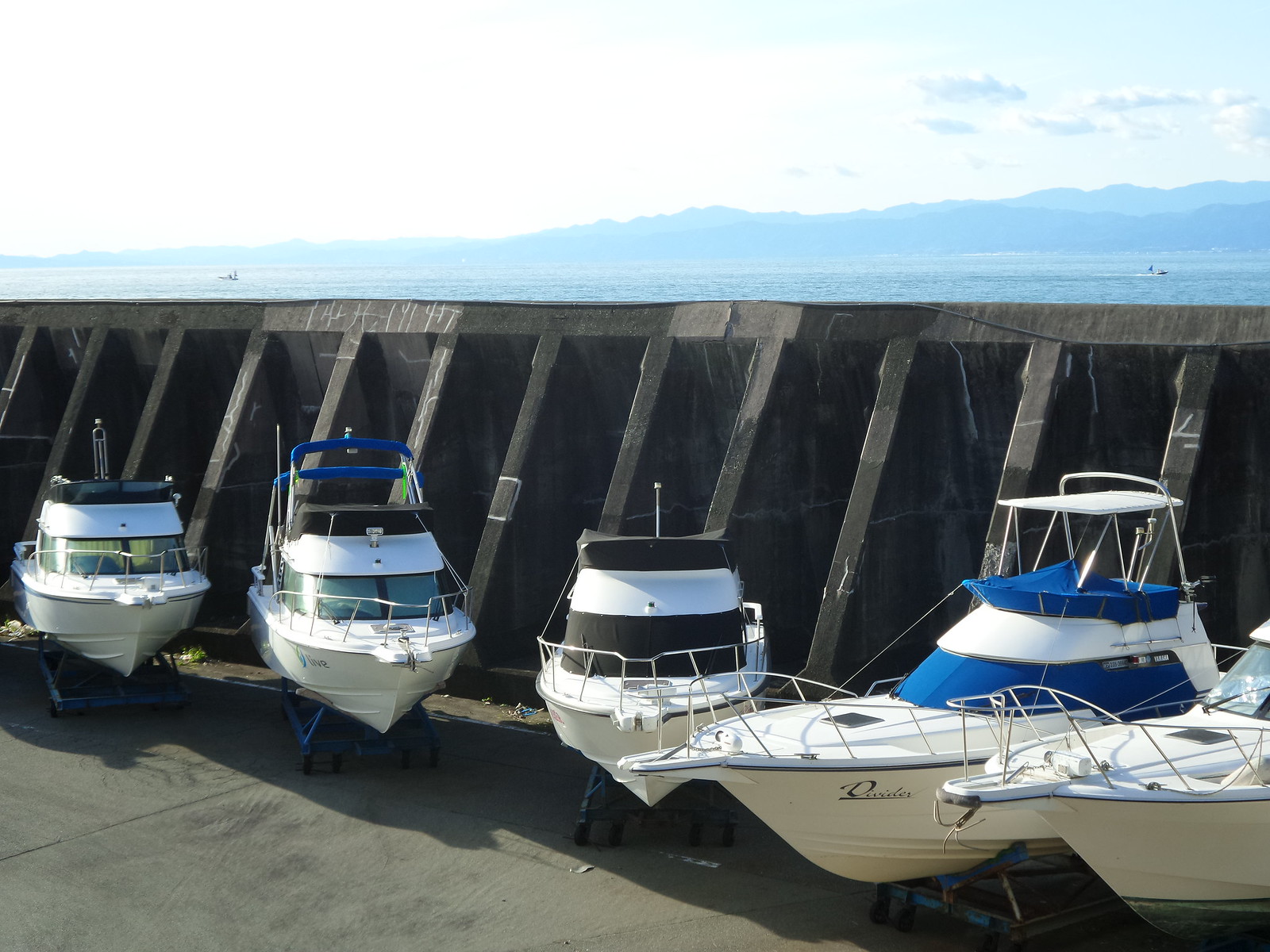In this detailed outdoor photograph, five white motorboats are stored on trailers in a boat yard against a rugged break wall. The boats, some adorned with blue, brown, and black accents, rest on a paved surface with traces of sand. Three boats are fully visible while two are partially cut off on the right side of the image. Above the break wall, the open sea gleams under a partly cloudy, gray sky. In the background, you can see bluish-colored mountains, and scattered boats are seen floating on the distant water. The entire scene captures a tranquil yet industrious marine atmosphere, framed in a rectangular composition.